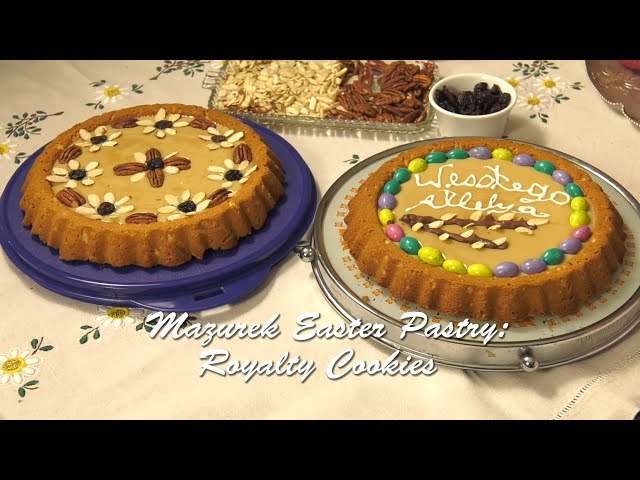The image showcases two elaborately decorated Easter pastries labeled "Mazurek Easter Pastry Royalty Cookies" in white italicized cursive at the bottom. Both pastries are large, circular cookies resembling an inverted Bundt cake, each filled and adorned with various ingredients. The cookie on the left is presented on a blue plastic serving tray and is embellished with pecans, peanuts, and raisins arranged to form floral patterns. The cookie on the right, set on a ceramic plate with a silver edge, is decorated with pastel-colored egg-shaped candies, forming a circular pattern around the text "Westigo Alea." A background tray contains assorted nuts, such as pecans and slivered almonds, alongside a small bowl of raisins or possibly peanut M&M's in Easter colors. The setting includes a daisy-patterned tablecloth.